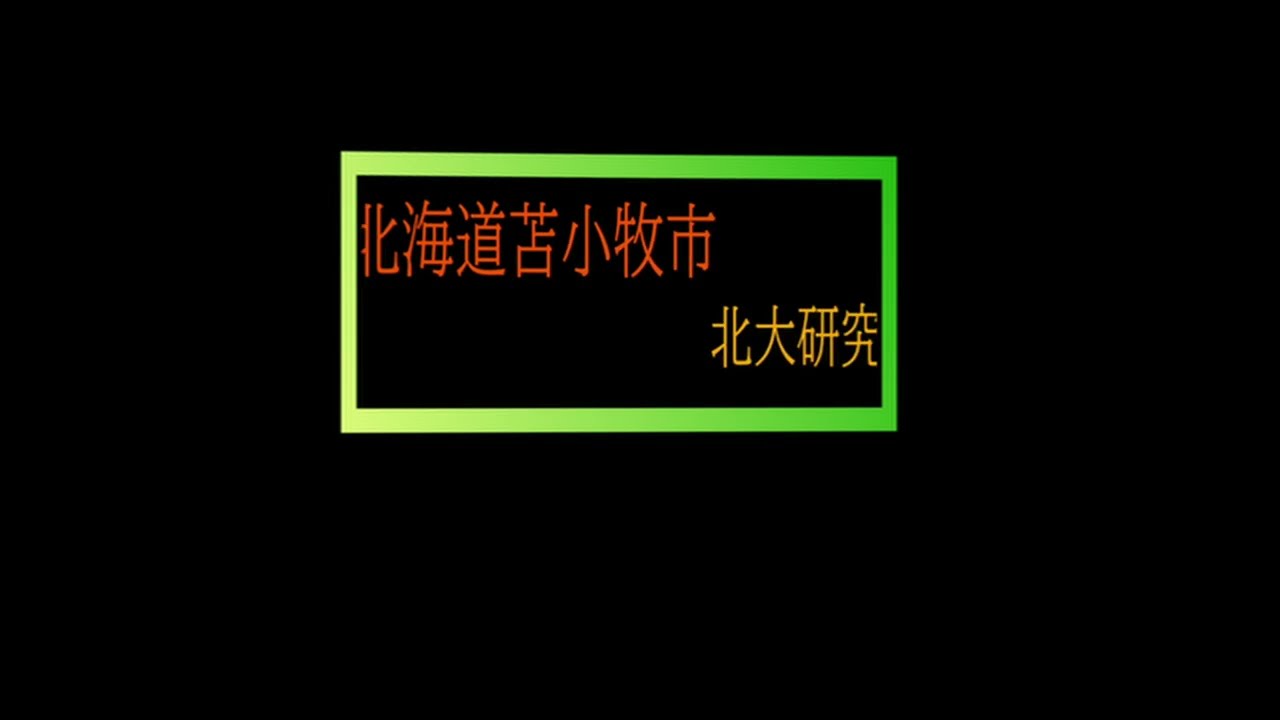The image features a predominantly black rectangle as its background. Centered within this dark expanse is a smaller, horizontally-oriented rectangle that transitions from a very light fluorescent green on the left to a dark fluorescent green on the right, creating an ombre effect. At the top edge of this green rectangle is a row of oriental characters in an orange font. Additionally, in the bottom right corner of the green rectangle, there is a smaller set of oriental characters in a yellow font. The entire scene is set against the stark contrast of the black background, making the neon green, orange, and yellow elements stand out vividly.